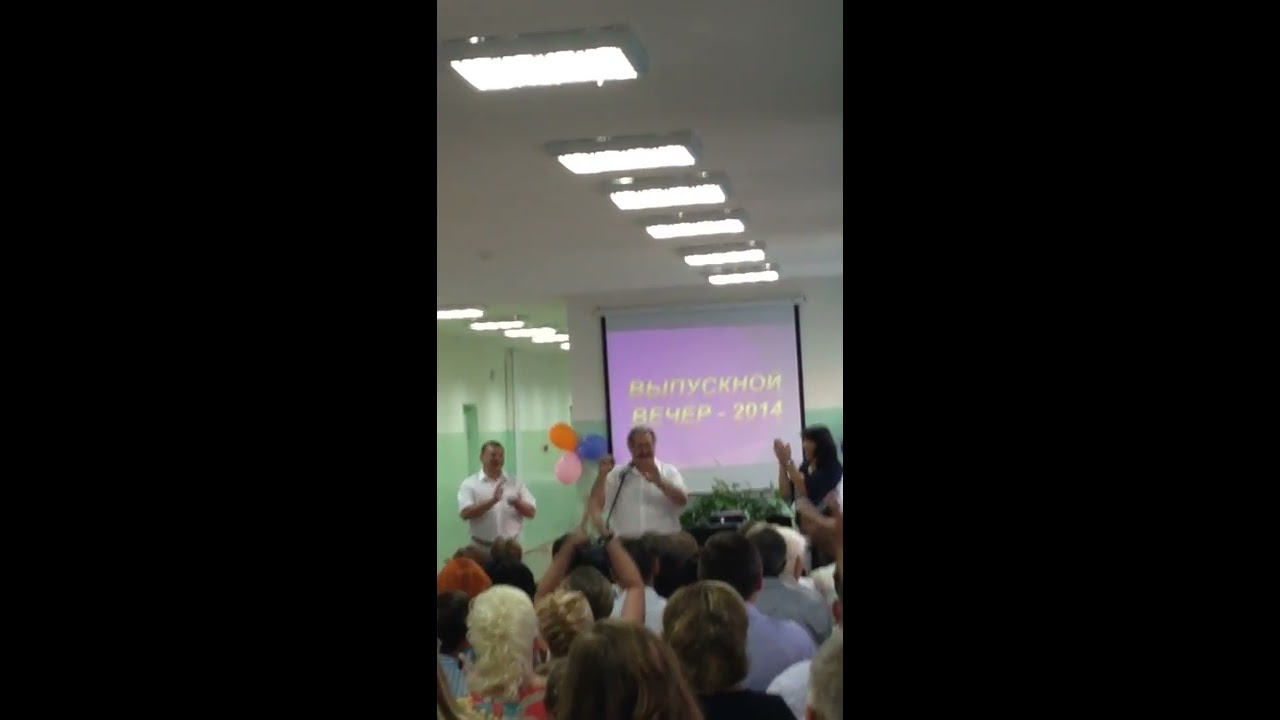The image depicts a slightly blurry and pixelated smartphone photograph, taken from a distance in portrait orientation over the heads of about 20 people gathered closely together. They are in what appears to be an office, classroom, or institutional setting with fluorescent ceiling lights. In the foreground, we see the varied hair colors of the attendees, including light brown, dark brown, and blonde, as they focus on two men at the front of the room. Both men are wearing white button-down shirts. One man is holding a microphone or a similar device to his mouth, appearing to speak, while the other is clapping. 

Behind them, a screen with a purple backdrop displays text in an unfamiliar language along with the year 2014 in yellow or white writing. The walls are painted in two tones of green or feature green tile work. Bright balloons in shades of orange, pink, and blue are taped to the wall beside the screen, adding a celebratory touch to the setting. The audience appears to be mixed-gender and formally dressed, lending the event a sense of importance.